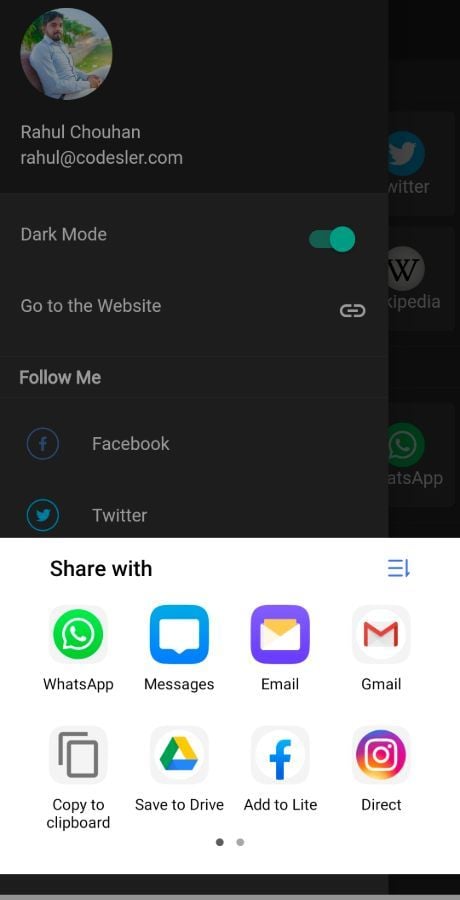This image is a detailed screenshot of an unknown website, likely a user profile or settings page. 

At the top left corner, within a circular frame, there's a profile picture of a man sitting on a bench. He is dressed in a light blue shirt paired with white pants and a black belt. He has dark black hair and a beard. Beneath the picture, the name "Rahul Chauhan" is prominently displayed, followed by his email address, "Rahul@Codelesser.com."

Immediately below the email, there is a section labeled "Dark Mode," accompanied by a greenish toggle button indicating that dark mode is currently enabled. 

Further down, there's an option labeled "Go to the Website," accompanied by a small paperclip icon on its right side. Under this option, there is a 'Follow Me' section, highlighting links to two social media platforms, Facebook and Twitter.

The bottom half of the image features various icons and logos categorized for different functions. The first row, labeled "Share," includes logos for WhatsApp, Messages, Email, and Gmail. Each of these logos is positioned above their respective labels. The second row contains options to "Copy to Clipboard," "Save to Drive," "Add to Light," and "Direct."

At the very bottom of the screenshot, there are two circular icons positioned in the bottom middle of the image. One circle is dark, while the one to the right is light red.